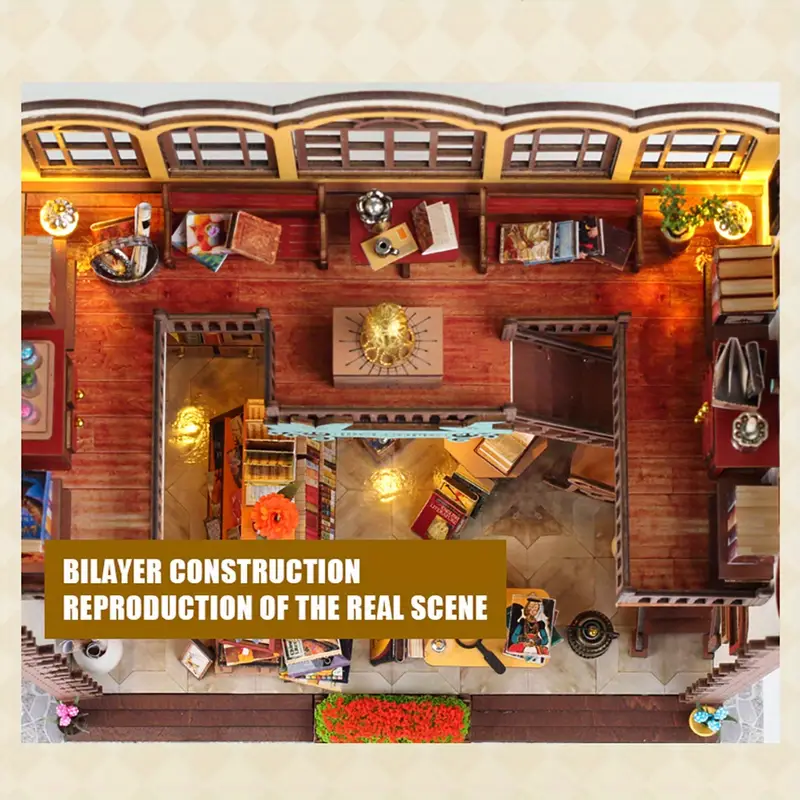The image showcases an overhead view of a meticulously detailed, vertically rectangular room that resembles a model or blueprint. The focal wall is adorned with a series of tall, arching windows framed in brown with yellow trim and white tops, allowing natural light to stream through. The dark reddish-brown hardwood floor is polished to a shine, adding warmth to the space. Central to the room is a light brown table embellished with a gold object, flanked by books and small plants adding a touch of greenery and life to the scene.

A staircase descends from the middle, leading to a second level with a lighter brown wooden floor, continuing the wood theme. The upper floor is lined with wood railings, cherry red hardwood, and a repeating pattern of shelving and cubbies, some filled with books, indicating a cozy reading nook. The walls are a warm yellow hue, complementing the overall aesthetic of the room. This space is illuminated by warm lights strategically placed in the upper left and upper right corners.

The image also includes a light brown rectangular label at the bottom that reads "Bilayer Construction, Reproduction of the Real Scene," signifying the conceptual nature of the depiction. Decorative red flowers add a final touch of vibrancy, making the room feel inviting and meticulously curated.